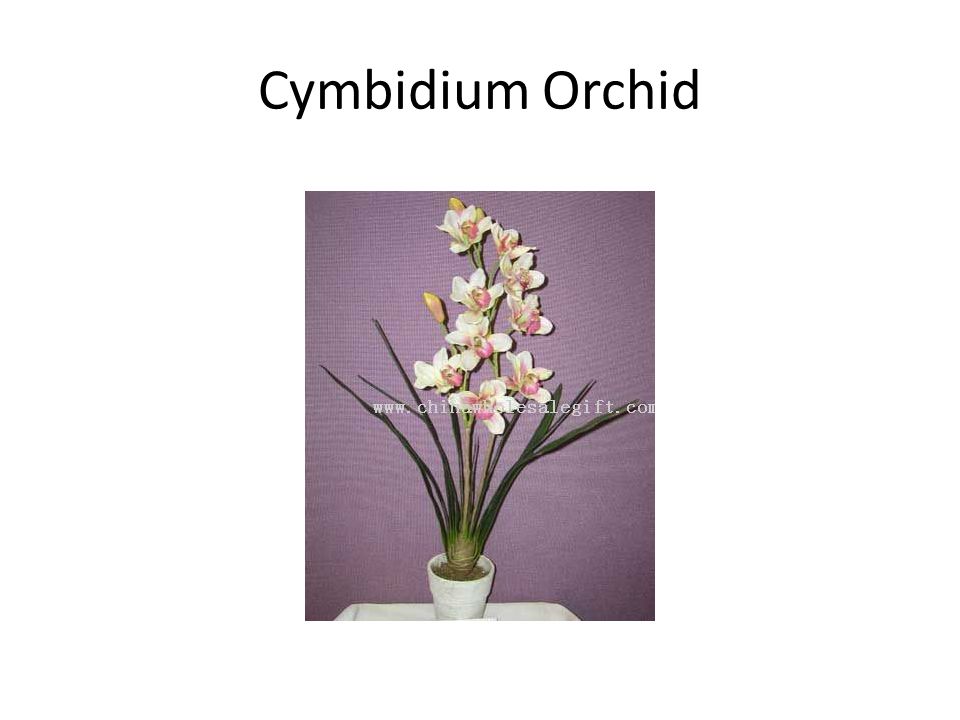The image features a lush Cymbidium orchid as the main focal point. The orchid is prominently centered in the picture, sitting in a smooth, white pot placed on a white table. The background is a textured, lilac purple, adding a stylish contrast to the greenery and the delicate petals of the plant. The orchid showcases a vibrant display of white, peach, light pink, and yellow-tinted blooms, accompanied by healthy green leaves strutting out from the base. The pot and table are only partially visible but clearly serve to elevate the beauty of the plant. Text at the top of the image reads "Cymbidium Orchid," and a small, white inscription www.chinawholesalegift.com overlays the flowers, subtly blending into the scene. The image captures a serene, decorative ambiance that could suit various settings, from personal hobbies to professional displays.